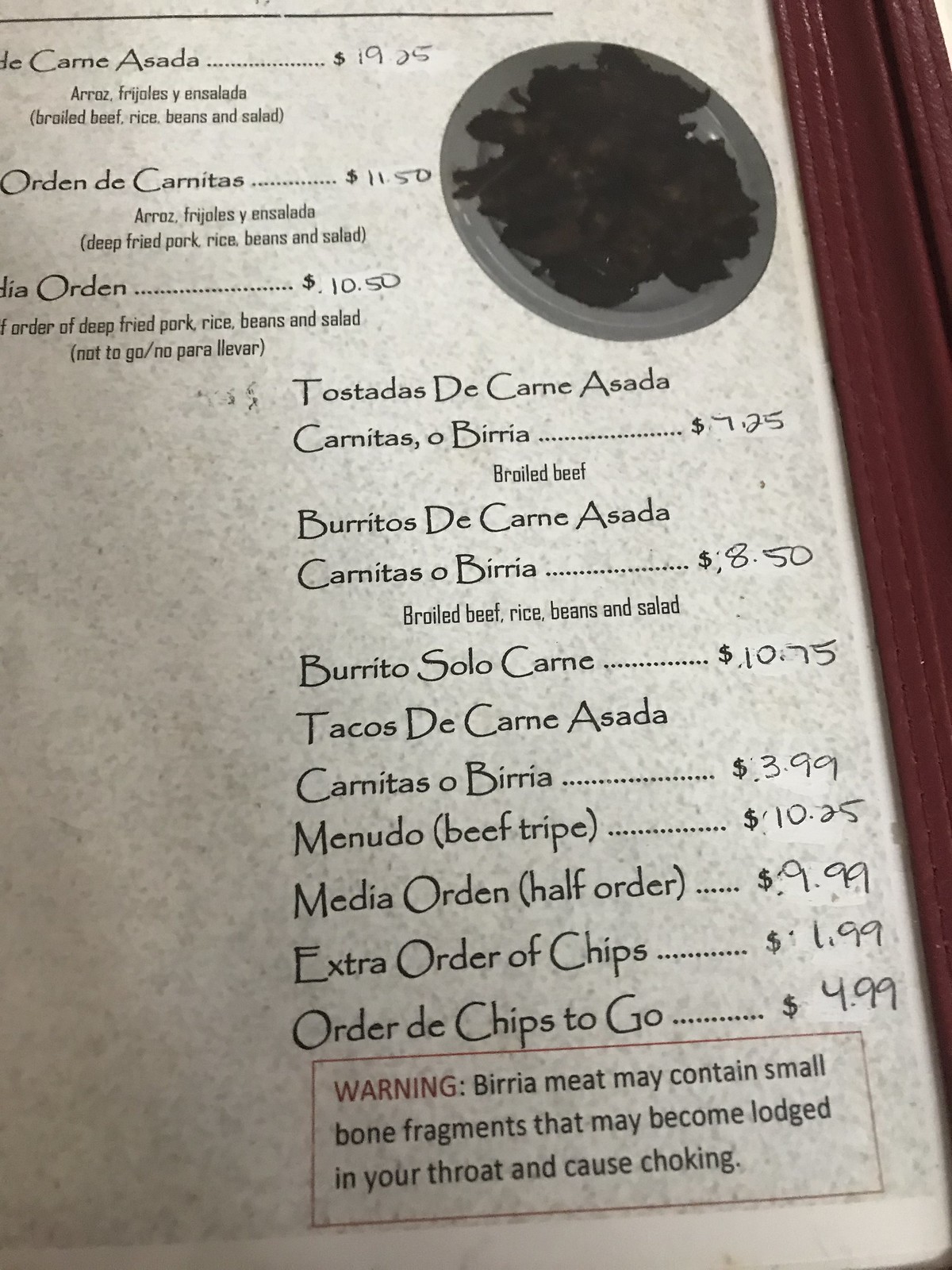This close-up photograph showcases an extensive menu presented in a dark brown vinyl binder. The vertical list of items is printed on light gray spackled paper using black ink, giving it a sophisticated yet straightforward appearance. Each dish is accompanied by detailed descriptions and corresponding prices, aligned to the right. Among the top-listed items are "Tostadas de Carne Asada," "Burrito Dishes," "Media Orden," and "Orden de Carnitas." Notably, at the bottom of the menu, there is a distinct warning enclosed in a box. The word "WARNING" is printed in red, followed by a cautionary message indicating that "Birria meat may contain small bone fragments that may become lodged in your throat and cause choking."